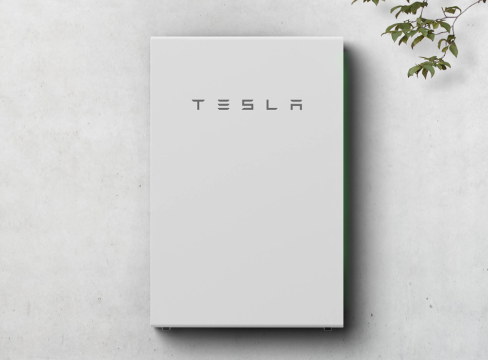This photograph features a minimalist, rectangular book set against a grayish, marble-like stone background. The background's subtle texture complements the book's whitish-gray cover, creating a seamless and almost camouflaged look. The composition is enhanced by the presence of delicate plant branches with small green leaves intruding from the upper right corner, adding a touch of natural elegance. Among these branches, only one is prominently visible, while the rest appear partially obscured, with a few leaves peeking in at the top.

The book, occupying approximately three-quarters of the photograph's vertical space, carries a simple yet striking design. Its surface is unadorned, save for the title "TESLA," engraved in capital letters at the top-center of the cover. The typography is distinctive; the letter "E" is fashioned from three horizontal lines, and the "A" lacks its usual connecting strokes, resulting in a blocky, geometric appearance. The title casts a subtle shadow, adding depth to the otherwise plain cover and drawing the viewer's attention to the central motif.

Overall, the image blends modern minimalism with natural elements, creating a serene and sophisticated composition centered around the enigmatic title "TESLA."